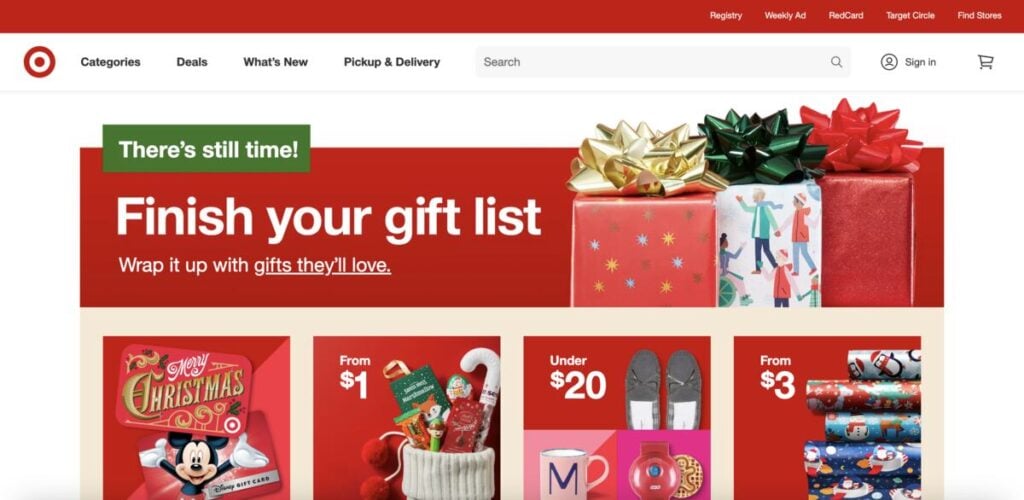The image appears to be a snapshot of a Target website. Dominating the top section is a distinctive red bar featuring white text aligned to the right. Prominently displayed on this bar is the Target logo accompanied by navigation options: "Categories," "Deals," "What's New," and "Pickup and Delivery." Below this bar lies a gray search rectangle positioned to the left, featuring a magnifying glass icon on its right side. Adjacent to this is a circular icon depicting a person, labeled "Sign In," alongside a shopping cart icon.

Beneath the navigation bar, a vibrant green rectangle catches the eye with text urging, "There's Still Time," while directly below, a red rectangle encourages visitors to "Finish Your Gift List." This red rectangle also features an underlined prompt, "Wrap it up with Gifts They'll Love."

To the right of these prompts is an image of three wrapped packages. Below this, a pinkish-red square showcases Mickey Mouse with a festive message reading "Happy Christmas." Next to this is another red square depicting the top of a Christmas stocking filled with items, labeled "From $1." Adjacent is a red rectangle highlighting a pair of slippers on its right side, and text on the left proclaiming "Under $20."

Further down, there’s an image of a mug situated to the left of another indistinguishable picture. Concluding the visual array, another red square displays text on the left that says "From $3" beside rolls of wrapping paper shown on the right.